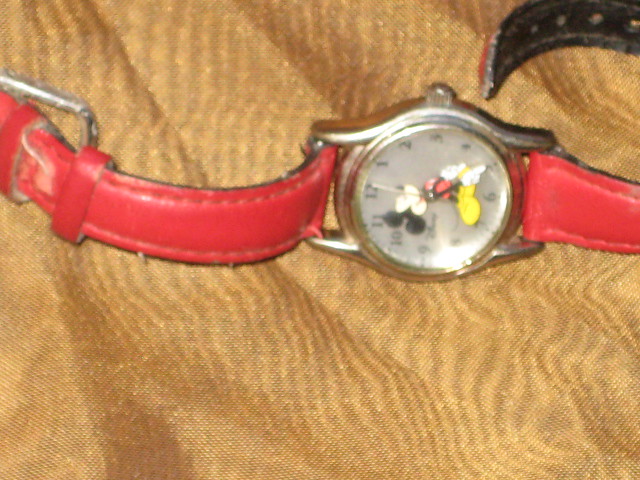This close-up image features a slightly blurry depiction of a classic Mickey Mouse watch resting on a beige cloth, possibly a bedspread. The watch has red leather straps and a silver bezel encircling its white face, which is marked by black numerals. On the watch face, an illustration of Mickey Mouse adds a playful touch. A small silver dial is visible on the right side of the watch. In the upper right-hand corner, the clasp of another watch is just discernible, hinting at the presence of a second timepiece nearby.